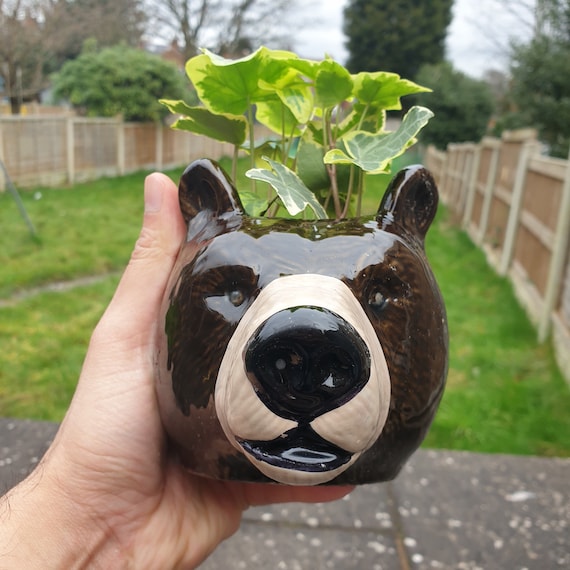The image captures a detailed and colorful photo of a fair-skinned man's hand, identifiable by some black hair on the wrist and a prominent thumb, holding up a small flower pot that resembles the size of a coffee mug. This pot is intricately designed to look like a bear's head, featuring a shiny brown coat, a large black nose surrounded by a light cream-colored muzzle, small black mouth, two little eyes, and distinct ears—resembling a mix between a brown or grizzly bear, though one description mentioned it looks like a black bear. Emerging from the top are small green ivy leaves or similarly small plants with green stalks and brown stems. The background reveals a typical backyard scene with green grass, trees with green leaves, a wooden fence on either side, and a slightly damp-looking concrete patio in the foreground.